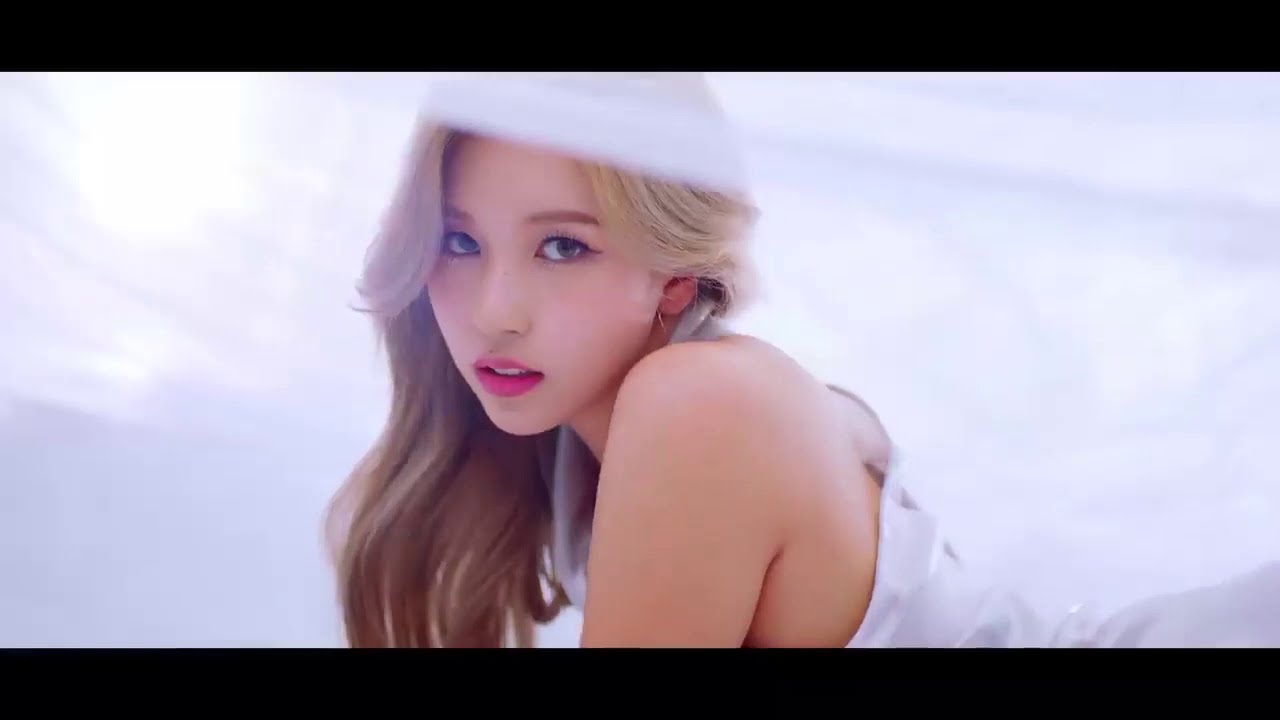In this image, a young Asian woman with long, dyed blonde hair is laying on her stomach surrounded by an ethereal, translucent white or silver backdrop. The image is framed with black borders at the top and bottom, giving it a cinematic feel as if it's a still from a music video. The woman's fair complexion is accentuated by her light blonde eyebrows and bright pink lipstick, with her lips slightly parted to reveal her teeth. She is propped up on her forearms, her bare left shoulder visible, and she's wearing a silky white outfit, possibly a halter top or a specific type of gown, that drapes elegantly over her. The soft light behind the sheer fabric casts an almost otherworldly glow over the scene, enhancing the dreamlike quality. Her blue contact lenses and sultry gaze directly into the camera add a layer of intensity to her serene yet captivating pose.